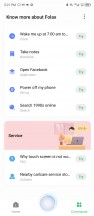This image appears to be a blurry, vertically-oriented screenshot likely captured from a phone. The screenshot includes the time displayed in the upper left corner, though the exact numbers are indiscernible—only the "PM" indicator is visible. The title at the top of the image is barely legible, reading something like “Know More About Folsom ________” with the second part being obscured or faint. Below the title, there are five icons listed along the left side with corresponding labels or descriptions next to each icon. Towards the bottom of the screenshot is a banner featuring a cartoon image of a man sitting at a desk adorned with flowers and an open laptop. This banner has a pink background, with text that seems to read "Service" alongside a bar.